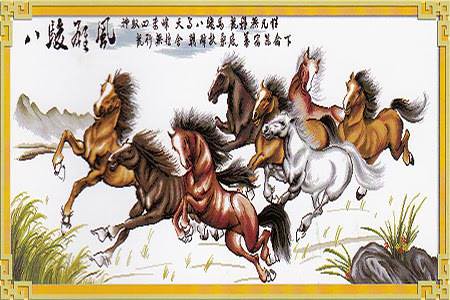A framed painting, encased in a gold frame with Asian design elements at each corner, depicts a dynamic scene of eight galloping horses. The horses, diverse in color with two dark brown, three light brown, one reddish, one dark ginger, and one white, are portrayed with wild manes, giving an impression of swift motion and untamed spirit. The white background is sparsely decorated with small patches of grass and shrubs, and to the left, towering mountains are faintly visible. At the top of the image, there is black text in a foreign language, rendered in two rows of Asian script. The artwork, created in a slightly cartoonish, Asian-inspired style, captures the essence of wild horses running free, devoid of saddles, and exuding a sense of freedom and vigor.